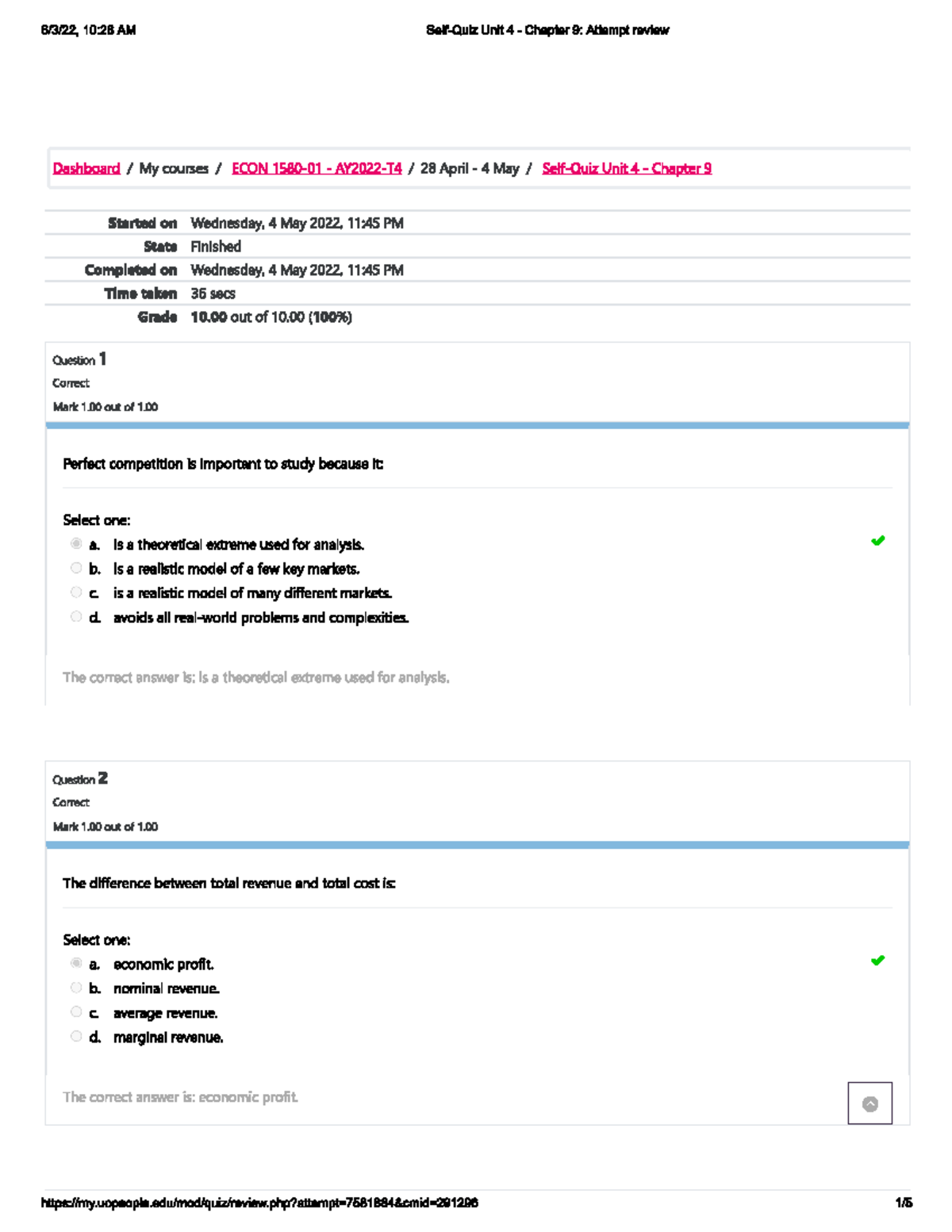The image displays a webpage titled "Self Quiz" at the top in small letters. It details an "Attempt Review" for Chapter 9. The webpage features a top navigation bar with "Dashboard" highlighted in red, alongside "My Courses." A red clickable link titled "ECON April 28th to May 4th Self Quiz Unit for Chapter 9" suggests the quiz pertains to economics.

Below this, the quiz details indicate it began and was completed on Wednesday, May 4, 2022, at 11:45 AM, with a total duration of 36 seconds. The quiz taker achieved a perfect score, earning 10 out of 10 points. 

Question 1, marked correct, inquires about the importance of perfect competition in study, followed by bullet points detailing various explanations. The correct answer, highlighted in gray, states it is "a theoretical extreme used for analysis."

Question 2, also correct and marked with 1 out of 1, asks about the difference between total revenue and total cost. It presents four multiple-choice options, labeled A, B, C, and D, requiring the user to select the correct one. The explanation in gray confirms the correct answer as "economic profit." 

In the lower right corner, there is a gray square with a circle icon. Beneath this icon, there's small, difficult-to-read black text, suggesting additional information might be present.